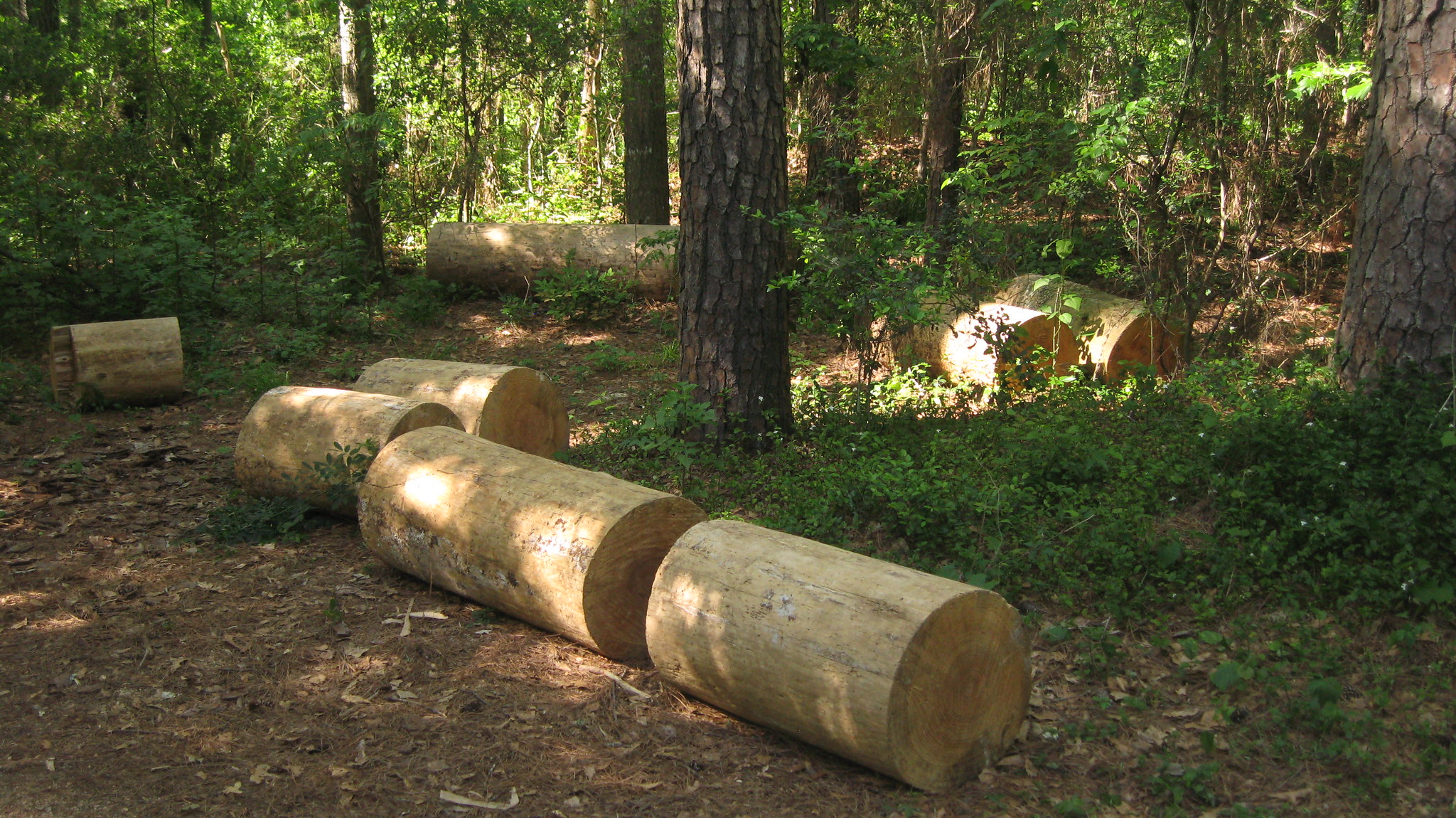The color photograph captures a serene, sunlit forest scene where a tree has been cut down into several neatly processed logs. The logs, which have been stripped of their bark, are cleanly cut and organized into multiple pieces, likely for a forestry project or lumber processing. There are at least eight sizable logs, each with a diameter of around two feet, lying on the forest floor amidst a carpet of fallen leaves and bare dirt. In the background, a tree stands tall with its trunk surrounded by lush green grass and additional smaller logs. A brown dirt path winds through the scene, leading towards the distant tree line accentuated with green foliage. The image conveys a peaceful yet industrious atmosphere, suggesting selective logging activities in a wooded, sun-dappled area.